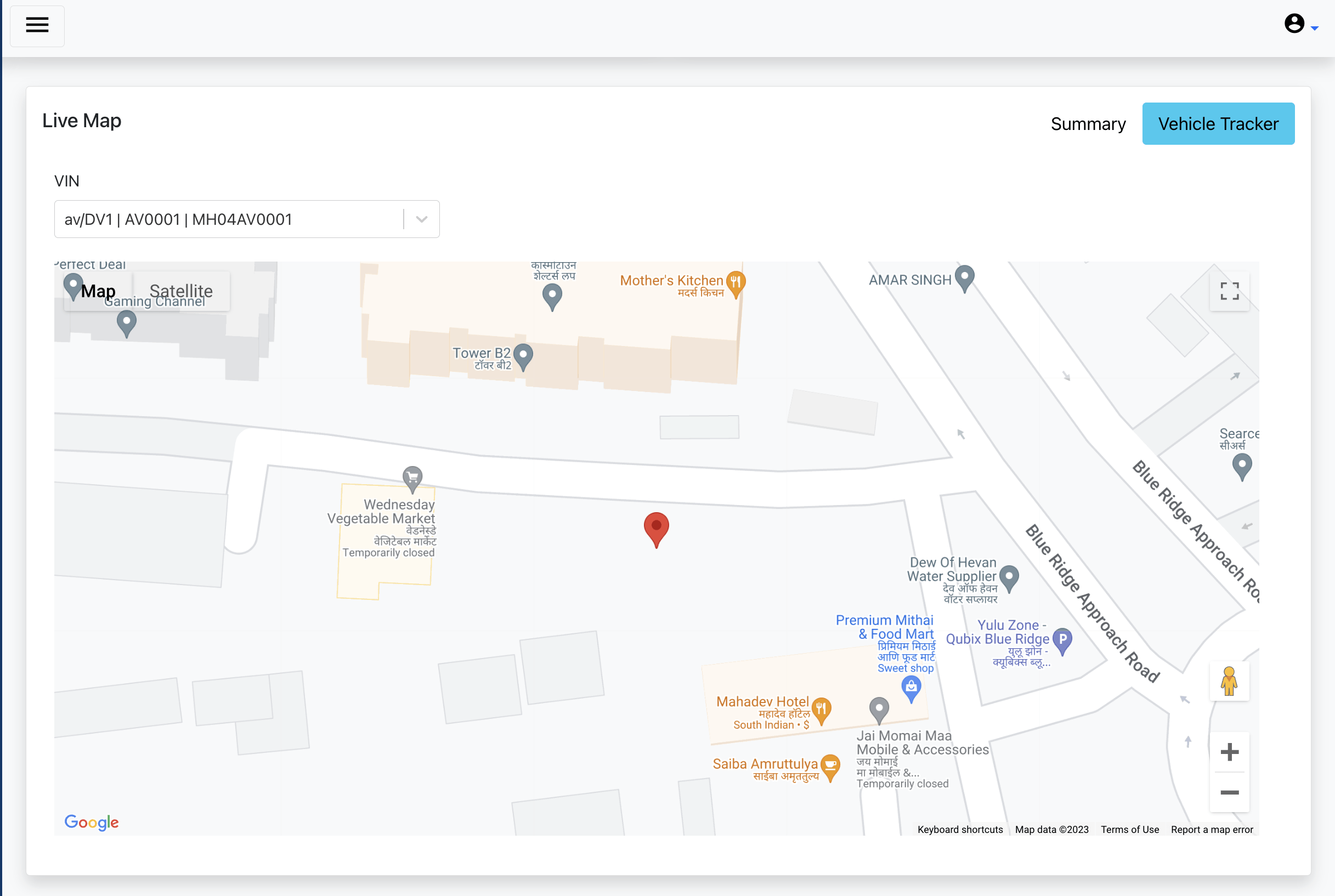This screenshot features a comprehensive live map interface set against a white background. In the top left-hand corner, there's a small drop-down menu. On the top right-hand corner, a user icon accompanied by a small arrow indicates another drop-down menu option. Below this, a prominent header spans the screen, with "Live Map" written on the left-hand side and a "Summary" label on the right. Adjacent to "Summary," a blue button labeled "Vehicle Tracker" is clearly visible.

On the left side of the display, there's a section labeled "VIN," underneath which lies a search bar containing various vehicle identification markers such as "av/dv1," "av0001," and "mh04av001." Below this VIN section, a detailed map is shown, displaying a street view punctuated by several marked locations. The Google logo is present in the lower left-hand corner, indicating the map data source. This carefully designed interface provides a comprehensive visual summary for tracking vehicle locations in real time.